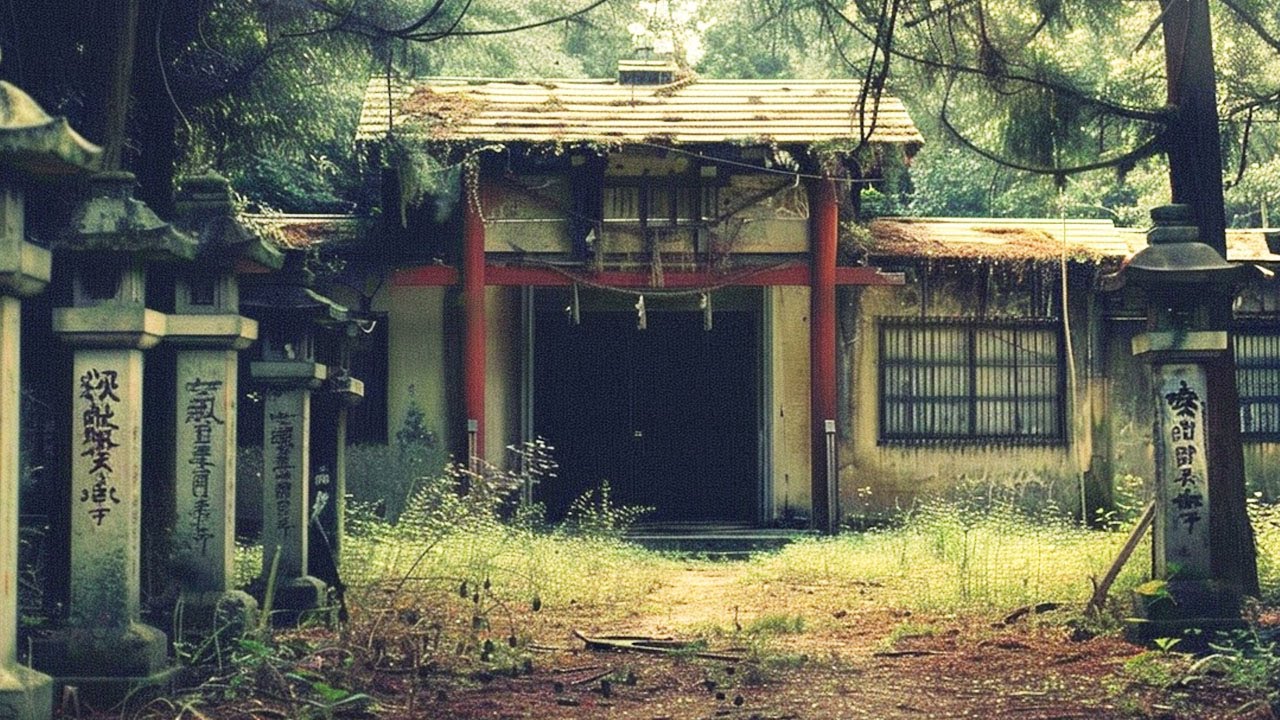This color photograph, wider than it is tall, showcases a dilapidated single-story building, possibly an ancient shrine of oriental design, surrounded by numerous trees and marked by overgrowth, including vines and tall, straggly grass. The structure appears to be made of cement with red supports, including two red pillars flanking a wide entryway topped by a horizontal red crossbar. Below this crossbar, two sacred ropes are tied between the pillars. The building features several stone lanterns and statues with vertical Chinese or Japanese characters inscribed on them, positioned on the left side of the image. The roof of the building is a brownish metal, and the windows are barred and closed. The foreground displays patchy grass with visible areas of brown dirt, adding to the sense of neglect surrounding this seemingly ancient site. There are no people visible in the photograph.